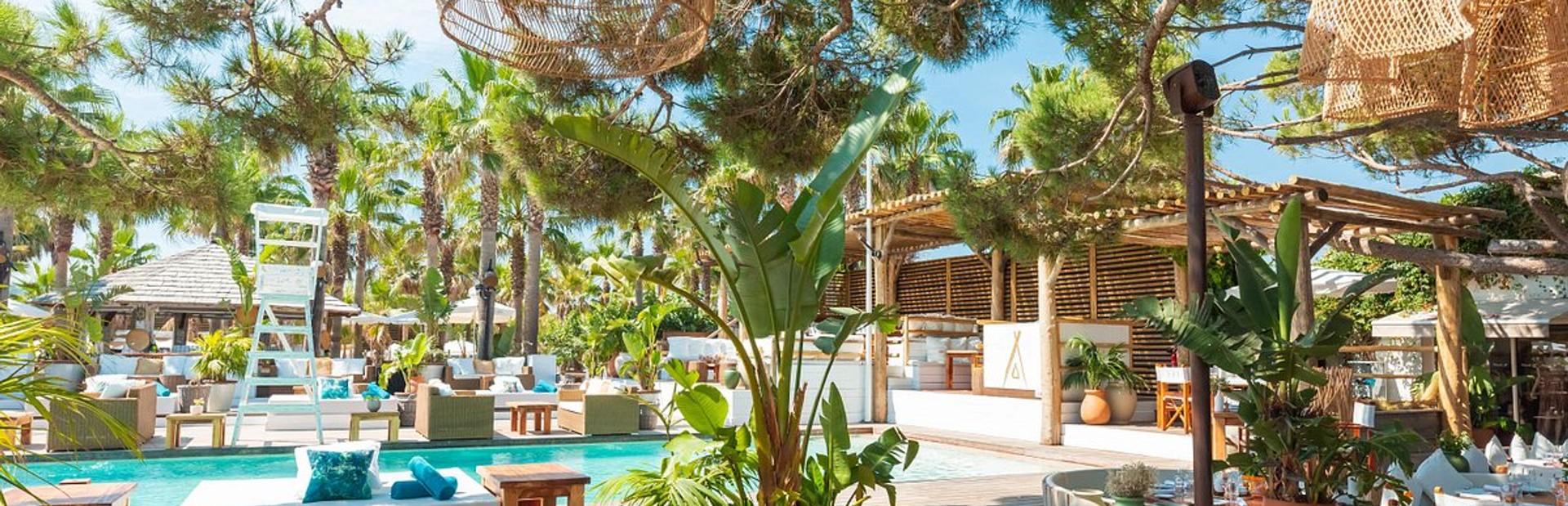This beautifully detailed image, likely a render due to its almost unreal vibrance, portrays a stunning outdoor poolside area. Central to the scene is a long, rectangular, bright bluish-green pool that sparkles invitingly. Surrounding the pool are several wicker benches and seating areas, as well as a white lifeguard tower positioned on the left side. The area is lush with various palm trees and other vividly colored foliage, adding an exotic feel to the environment. 

On the right side, you'll find a wooden pergola with a seating section beneath it, complemented by hanging wicker baskets and shades. Behind the pergola stands a wooden wall adorned with potted plants. Additionally, there's another roofed shelter towards the back. The sky is a clear, deep blue, enhancing the idyllic atmosphere of this luxurious outdoor space.